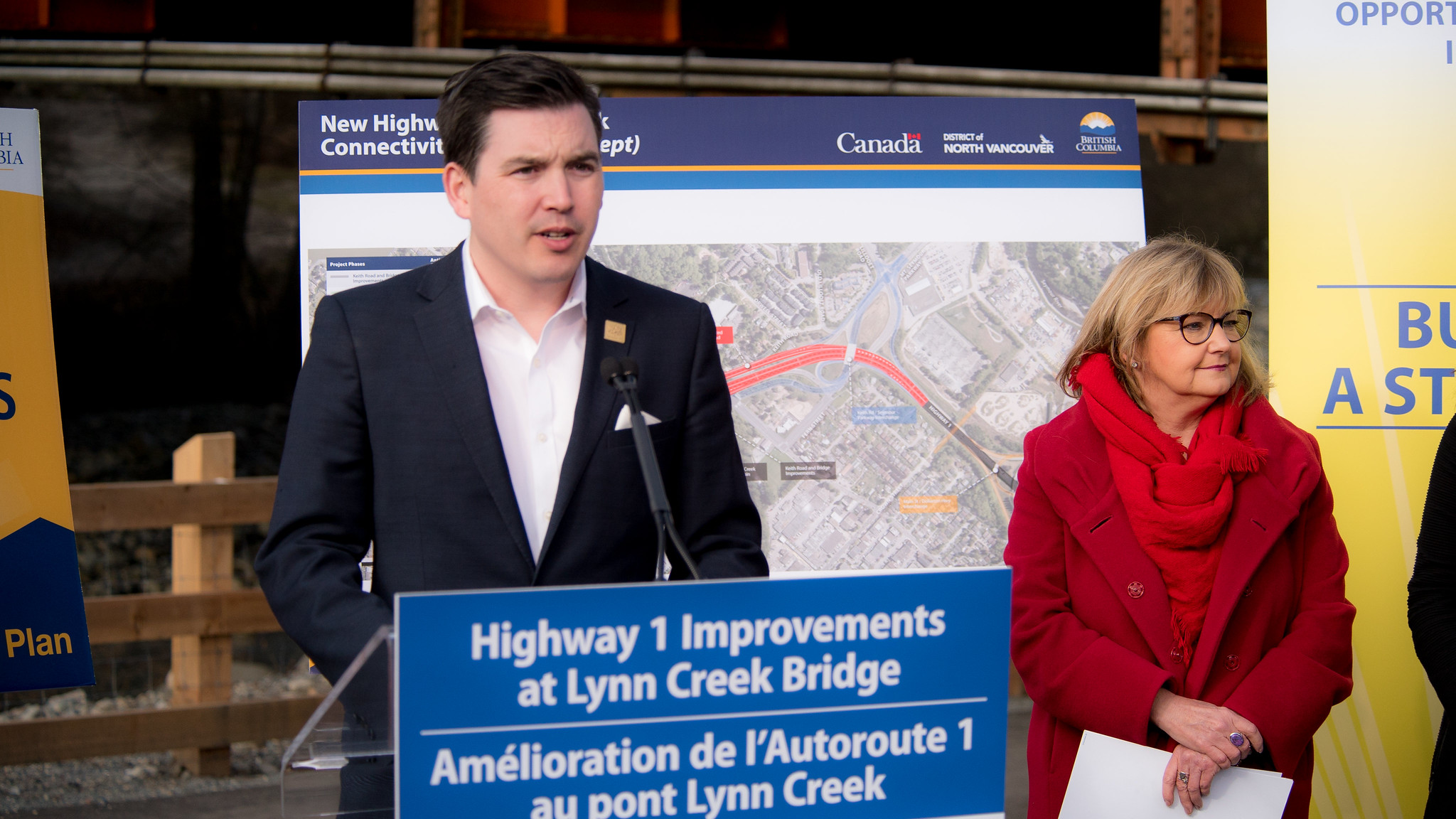In the image, a man and a woman are standing at a podium outdoors, likely in Canada, as suggested by the bilingual English and French text. The man, a Caucasian with short dark hair, is dressed in a white dress shirt and a navy blue blazer. He appears to be giving a serious speech at the podium, which displays a blue sign with white text reading "Highway One Improvements at Lynn Creek Bridge," followed by the French translation. Beside him stands a woman, possibly in her 50s, with blonde hair and bangs, wearing black glasses, a heavy red coat, and a red scarf. She seems to be holding a white paper and appears involved in the project. Both are positioned in front of a large map highlighting the highways, including the areas of planned improvements, indicated by colored lines. To their side, yellow banners or billboards are partially visible, hinting at additional information related to the event.